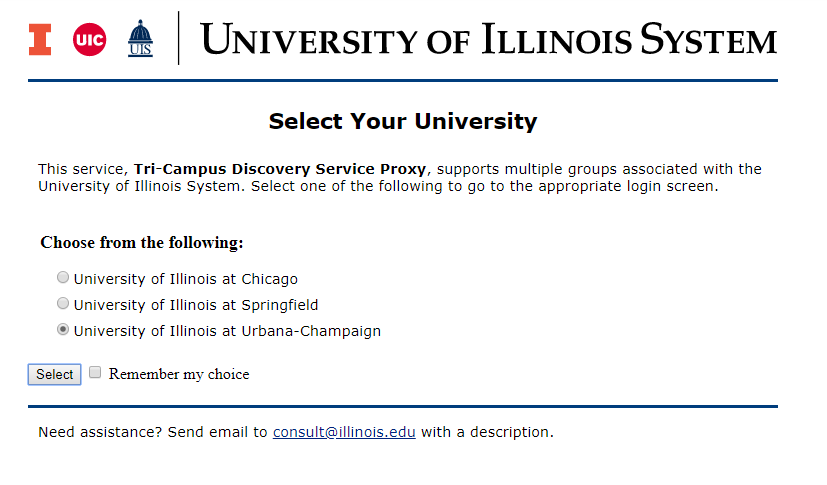This screenshot depicts the desktop view of a University of Illinois System login portal. At the top left corner, an orange "I" is prominently displayed alongside a red circle with white text that reads "UIC." Adjacent to this, there is an icon resembling either a bell or a person wearing a ball gown, followed by the text "UIC" again. Beneath these icons, a dividing line separates them from the next section of content.

In bold, all-capital text, the words "UNIVERSITY OF ILLINOIS SYSTEM" are displayed, followed by another horizontal line. Below this, bold text instructs the user to "SELECT YOUR UNIVERSITY." The subsequent section explains, in regular text, that the service—bolded as "Tri-Campus Discovery Service Proxy"—supports multiple groups affiliated with the University of Illinois System. Users are prompted to select one of the options to proceed to the appropriate login screen.

In bold text, users are advised to "CHOOSE FROM THE FOLLOWING," which is followed by three radio buttons. The options listed are:

1. University of Illinois at Chicago
2. University of Illinois at Springfield
3. University of Illinois at Urbana-Champaign (currently selected)

Each option has an adjacent "Select" button where users can confirm their choice, and a checkbox to "Remember my choice." At the very bottom, there is a note stating, "Need assistance? Send email to consult at illinois.edu with a description," indicating where users can seek help if required. This portal clearly serves as a gateway to access different University of Illinois campuses depending on the user's affiliation.